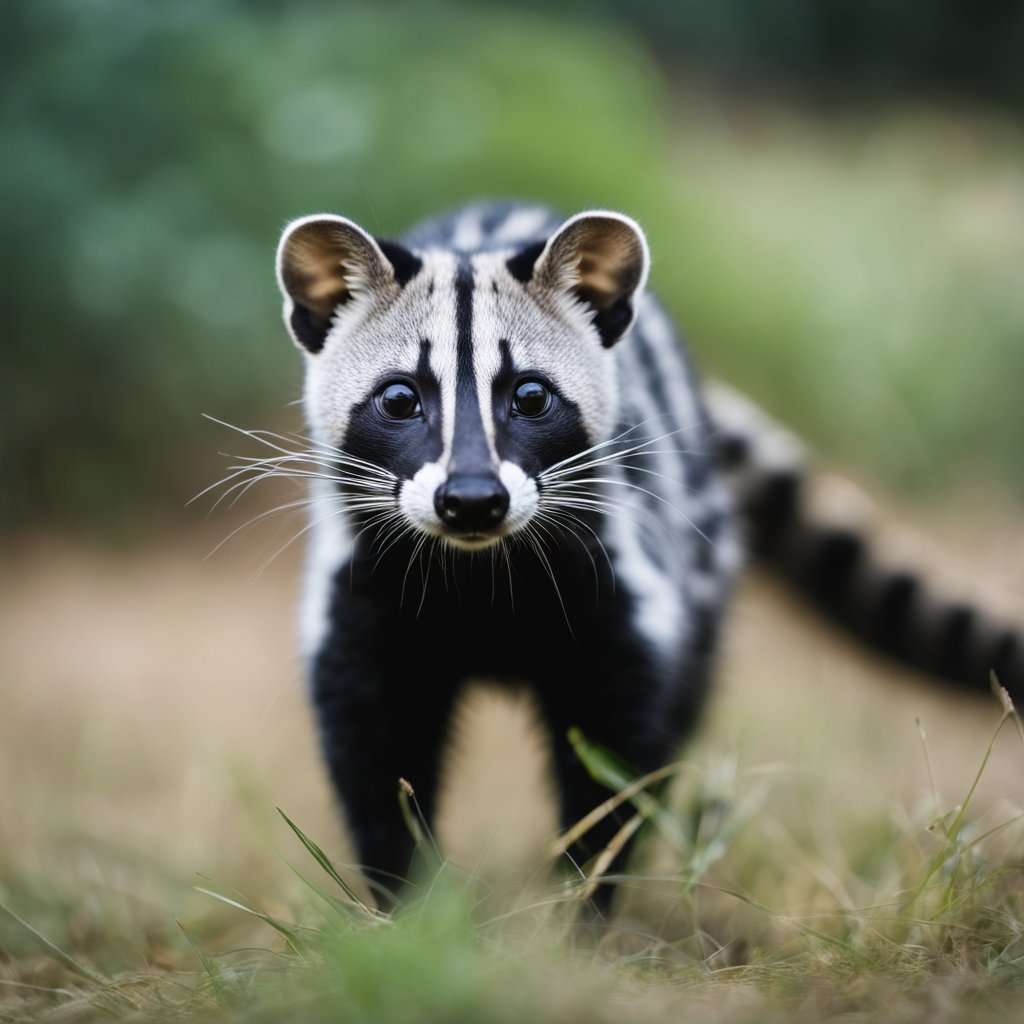The photograph captures a close-up of a serval in an outdoor setting, though the background of greenery and brown dirt is blurred, giving a hint of its natural habitat. In the foreground, some pieces of grass are in focus, adding to the natural environment. The serval is looking directly at the camera, showcasing its striking facial features. It has dark black eyes, a round black nose, and white whiskers protruding to the sides. The serval's face features distinctive black markings around its eyes and a black stripe running from its nose to its forehead, resembling a raccoon. Its fur has a mixture of light brown tan and black striping and streaks, with its black and white tail visible but somewhat blurred. The legs of the serval are entirely black, providing a stark contrast to its predominantly lighter fur. The serval’s ears are large, round, and upright, adding to its keen, alert appearance.